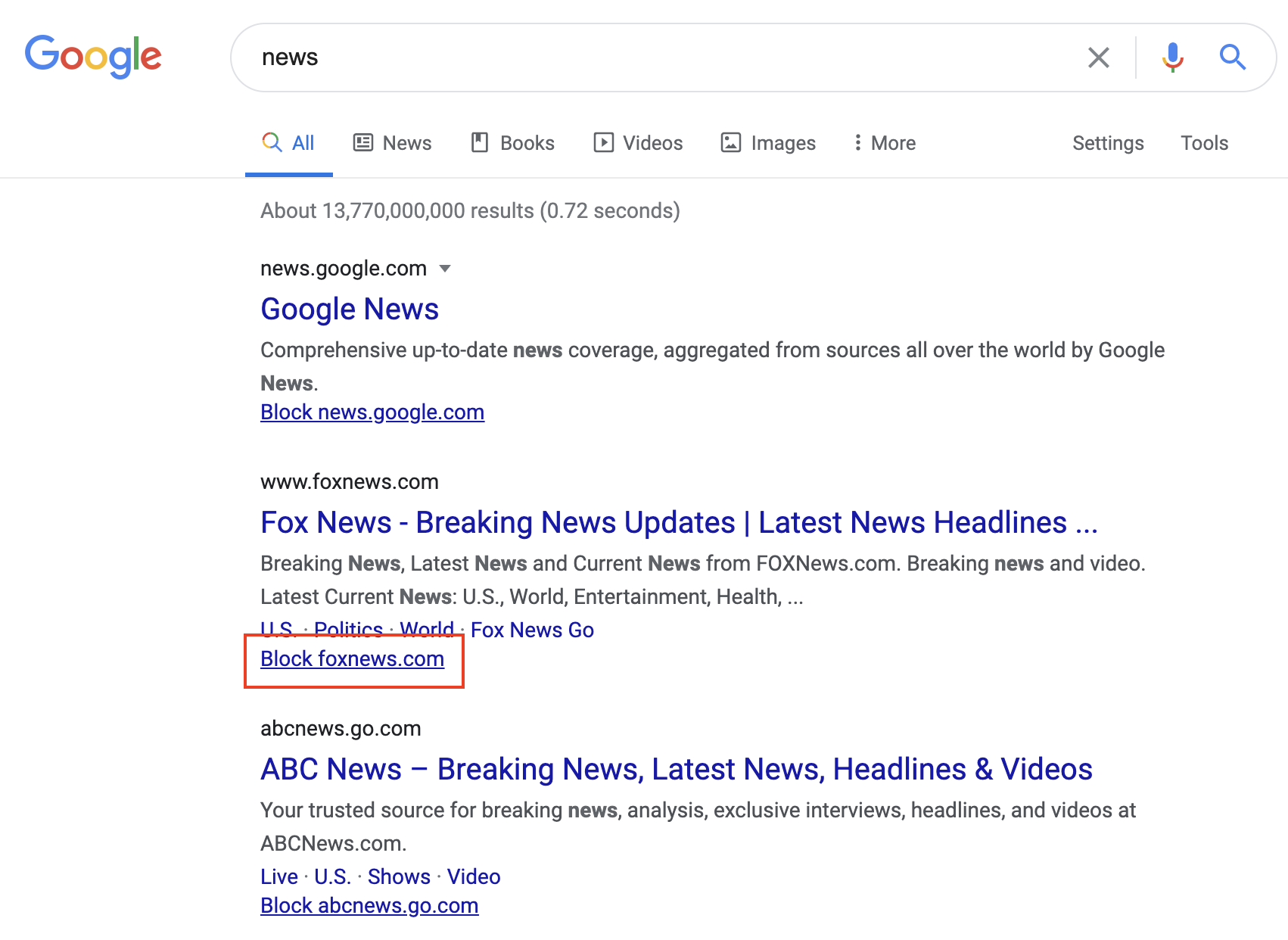This image is a cropped screenshot of a Google search with the distinctive Google logo visible in the top left corner. The search bar, positioned to the right of the logo, has the term "News" entered as the query. Below the search bar, the search results are arranged in a vertical list.

The first search result is for Google News, identified by the URL "news.google.com." The text "Google News" is prominently displayed in bold blue font. Directly underneath, there is a hyperlink "block.googlenews.com" shown in blue underlined text.

The second search result is for Fox News, with "Fox News breaking news updates, latest news headlines" similarly presented in bold blue font. Beneath this is a descriptive snippet of the site’s content. A hyperlink, "block.foxnews.com," appears at the bottom in blue underlined text. This entry is highlighted with a red box edited around the "block.foxnews.com" hyperlink, indicating that this is the link to block Fox News from appearing in the browser or search results.

The final visible search result is for ABC News, with "ABC News breaking news latest news headlines and videos" also presented in blue font. Just below it, there is a brief description of the site's content, followed by the website link "abcnews.go.com."

Overall, the screenshot clearly displays the top three search results for the query "News," with an added visual cue in the form of a red box to highlight the blocking option for Fox News.